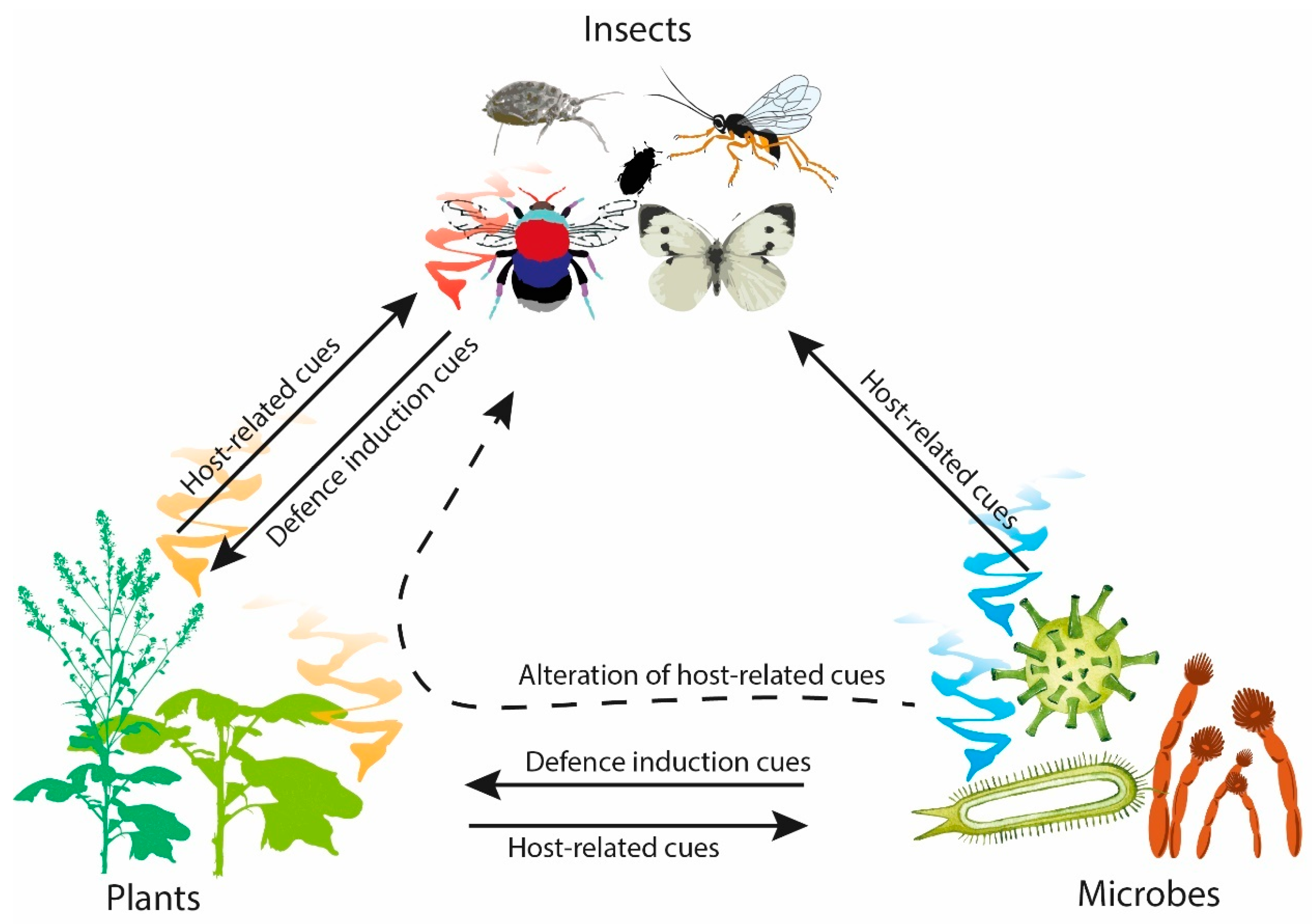This is a detailed scientific diagram illustrating the complex interactions between insects, plants, and microbes, forming a triangular flowchart. At the top, labeled "insects" in black text, there are detailed images of various insects including a bee, beetle, wasp, and butterfly. The lower right corner, labeled "microbes," depicts colorful microbes such as a spiky green sphere, blue spirals, a green paramecium-like organism with multiple legs and antennae, and reddish-orange anemone-like structures. The bottom left corner is labeled "plants," showing several green plants.

The diagram features several arrows with specific labels demonstrating the interactions:
- Arrows from "microbes" to both "insects" and "plants" are labeled "host-related cues."
- An arrow from "plants" to "insects" also reads "host-related cues."
- From "insects" to "plants" there's an arrow labeled "defense induction cues."
- Arrows between "plants" and "microbes" are labeled reciprocally with "host-related cues" and "defense induction cues."
- Additionally, a dotted arrow from "microbes" to "insects" is labeled "alteration of host-related cues."

This intricate diagram visually represents how these organisms interact through various biochemical signals and defense mechanisms.